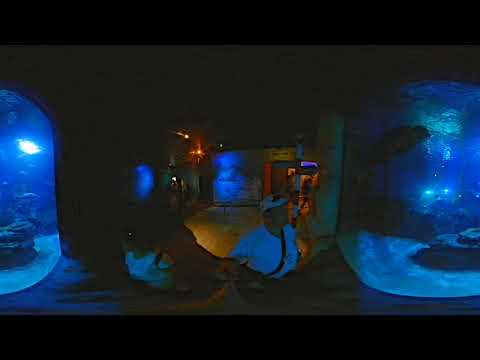This detailed panoramic vertical image, likely captured using 360 imaging, depicts a very dark scene, either at nighttime or within a dimly lit indoor aquarium. The image is bordered by black horizontal stripes at the top and bottom, emphasizing its central content. On either side of the picture, there appear to be large light blue jugs or small aquariums containing rocks. In the center, two people are visible, predominantly showing their upper bodies. One person, wearing a light-colored shirt and hat, walks toward the right. Another individual is partially visible near the lower left. The background features subdued blue lighting and grayish-green walls adorned with indistinct objects, possibly adding to the underwater ambiance. Although details are murky, hints of water and rocks are noticeable, but no fish are clearly visible, contributing to the enigmatic nature of the scene.